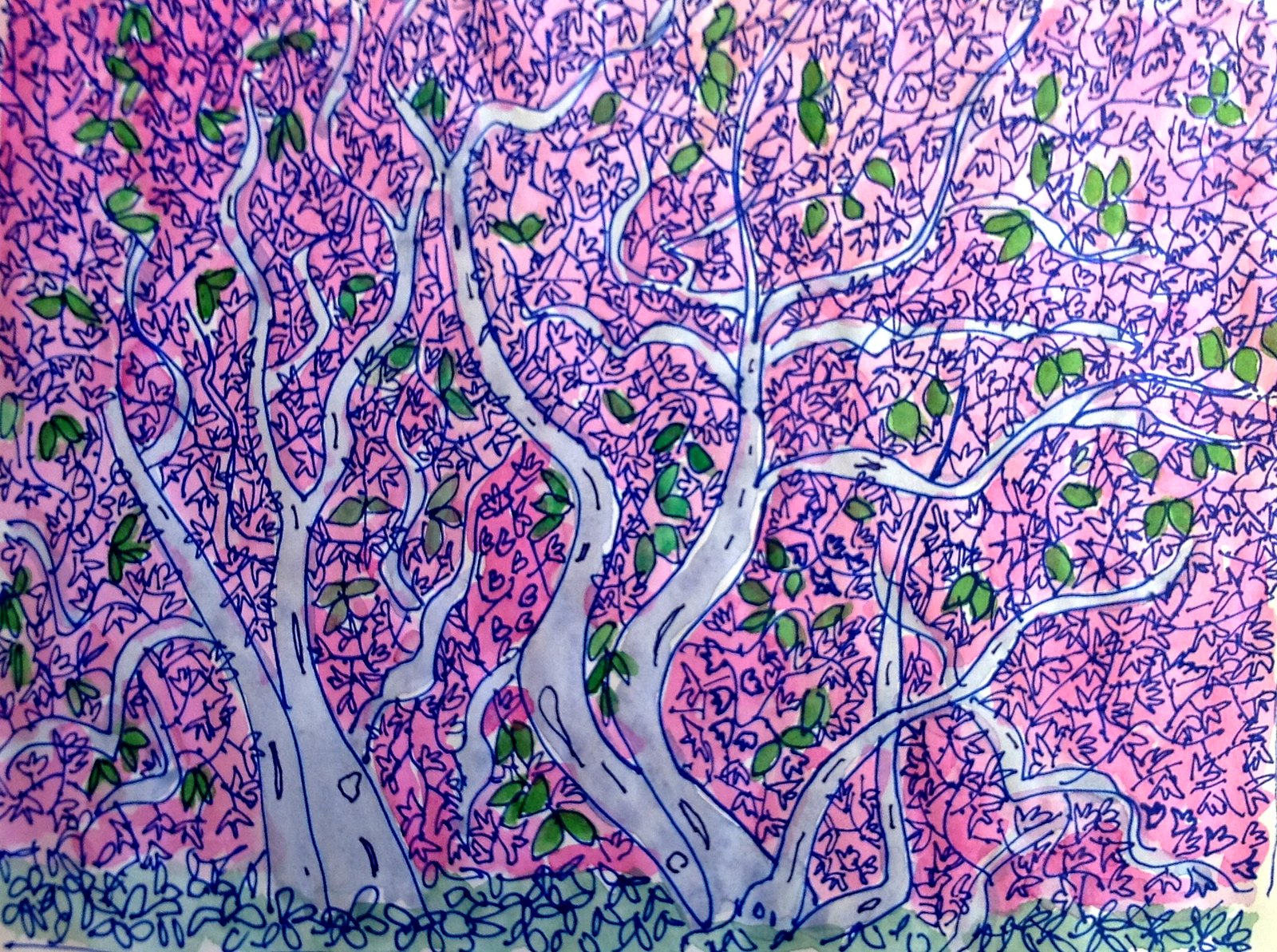This artwork is a densely drawn illustration that combines watercolor and blue ink line art, potentially created with a felt tip marker or ballpoint pen. The scene is filled with tightly packed lines and minimal white spaces, depicting two prominent clumps of trees with light gray trunks and branches. The trees exhibit sparse, small leaves that have a greenish hue with yellow undertones. 

The background of the piece is predominantly pink, transitioning from darker shades in the lower center to lighter hues in the upper right-hand corner. Along the bottom edge of the illustration, there is a strip of pale green foliage, outlined in blue, showcasing either flowers or leaves. The overall style is reminiscent of a child's doodle but with sophisticated detailing and technique, giving the image a whimsical yet intricate appearance.